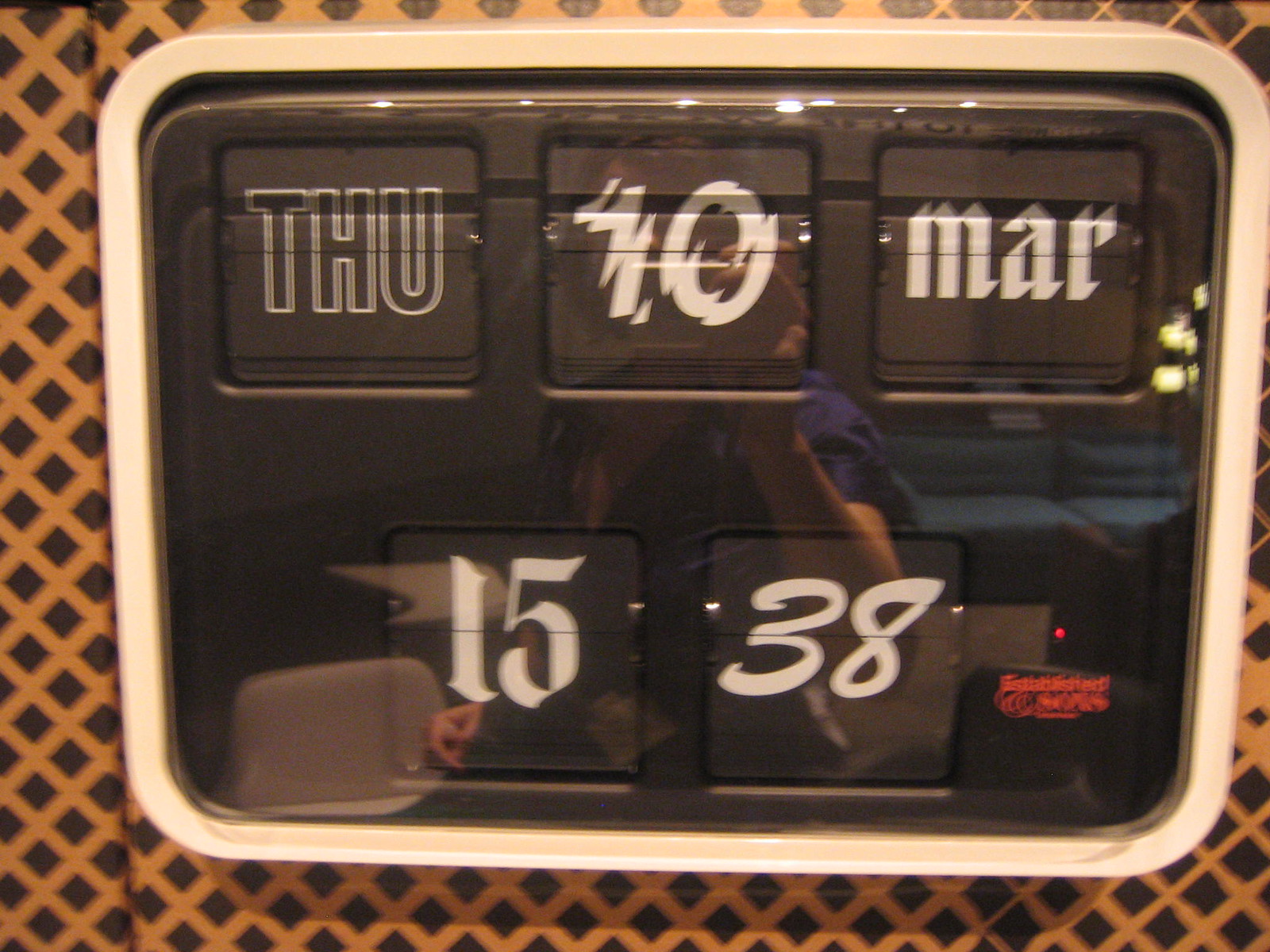The photo displays a black electronic calendar embedded in an off-white, rectangular frame with curved corners. The calendar is set against a wall or patterned wallpaper featuring black diamonds and orange-brown diamond-shaped hatching. The device prominently shows "THU" for Thursday in the top left slot, "10" in the center, and "MAR" for March on the top right. Below, the time is indicated as "1538" in 24-hour format, which translates to 3:38 PM. In the bottom left slot, it displays the date "15". A red logo, indistinct but visible, is located on the bottom right against the black background. Reflecting on the glass surface of the calendar is the person taking the picture, identifiable by their blue shirt and hands holding a phone. Behind the person, there are chairs and possibly a blue couch or lounge furniture.